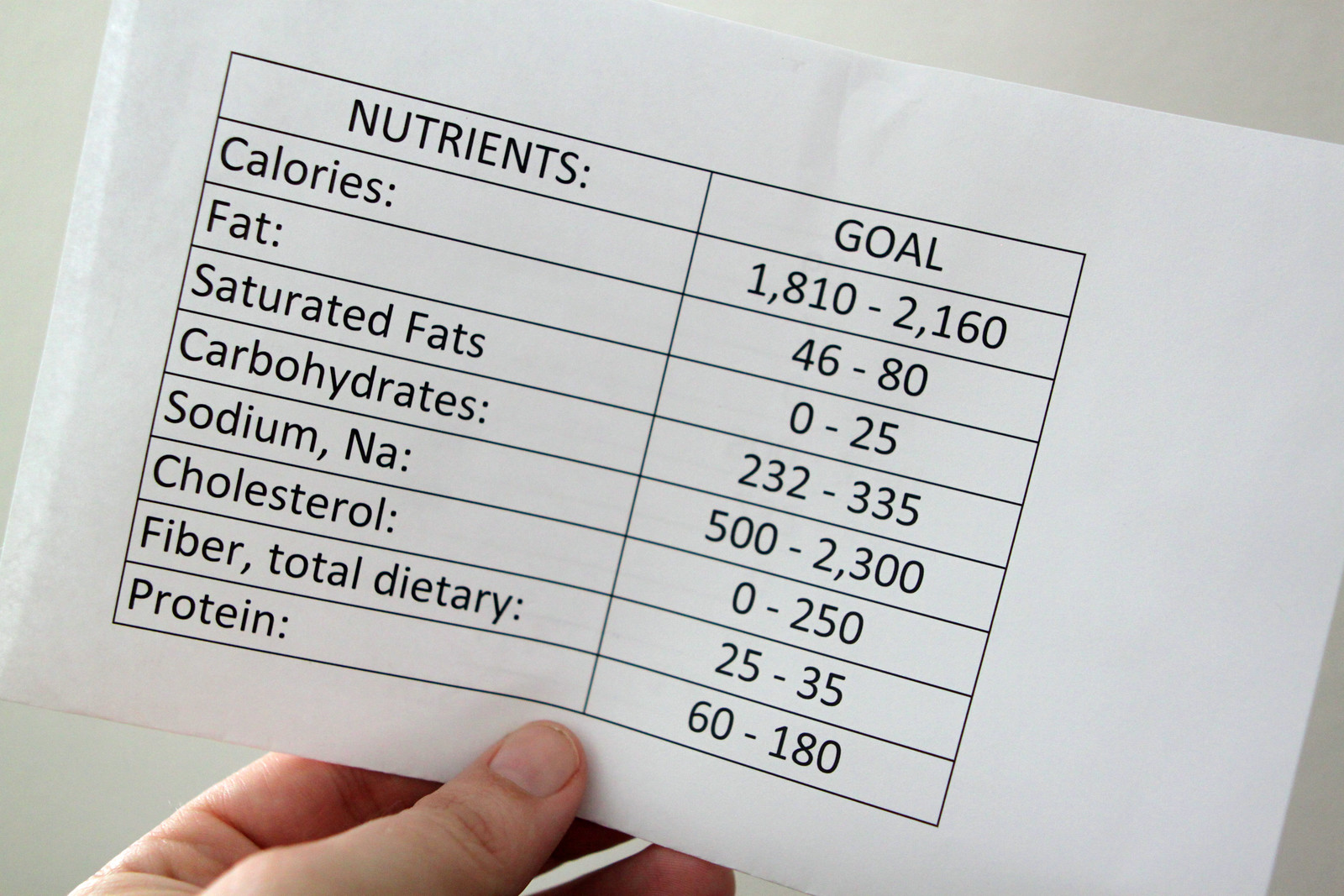In this image, a hand is prominently featured at the bottom, primarily showing the top of the thumb. The hand is holding a white piece of paper that is slightly folded. The paper is printed with black text organized into two distinct columns, each containing nine rows of information. The left column is titled "Nutrients" and lists various nutritional components: Calories, Fat, Saturated Fats, Carbohydrates, Sodium, NA, Cholesterol, Fiber, Total Dietary, and Protein. The right column, titled "Goal," specifies target ranges for each nutrient respectively: 1810 to 2160, 46 to 80, 0 to 25, 232 to 335, 500 to 2300, 0 to 250, 25 to 35, and 60 to 180. The background of the image is plain white, providing a stark contrast that highlights the text and the hand holding the paper.